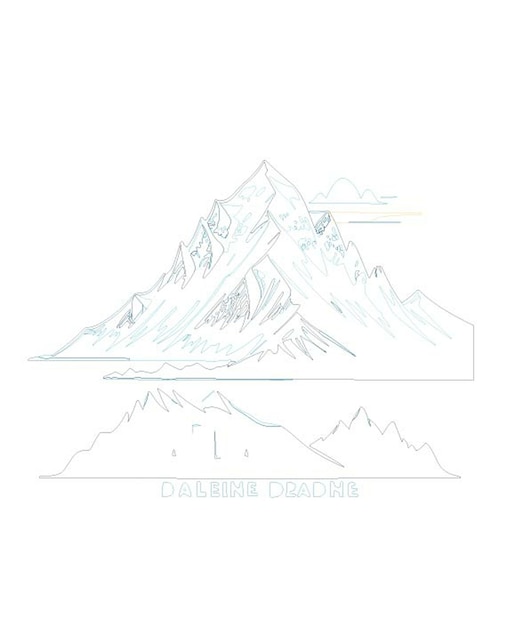The artwork features two distinct yet related sketches of mountains drawn primarily with colored pencils in light gray and turquoise blue. The upper sketch is more detailed, showcasing mountains with textured slopes, possibly snow at the peaks, and abstract representations of clouds and a sun in the background—highlighted by a pale yellow stripe. The shading varies, with some darker areas indicating where more pressure was applied. The lower sketch is much simpler, almost an outline, with minimal interior detail, resembling another view of the mountain from the first sketch or an adjacent peak. Below the sketches, in light pencil and capital letters, is the inscription "Dahline, D-A-L-E-I-N-E, Dradhe, D-R-A-D-H-E," which is presumably the artist's name.